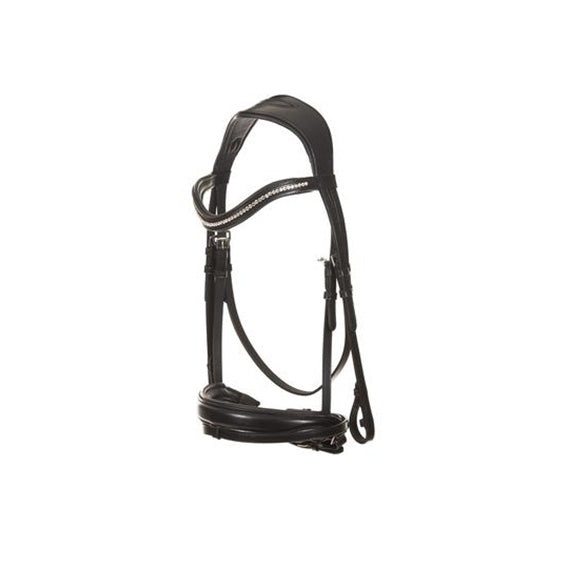The image depicts a black-colored leather bridle, possibly for a horse, set against a white background. The bridle is compactly folded, causing it to overlap and obscure certain details. The black leather is accented with silver buckles on the left and right sides. A black strap with a white line is visibly part of the bridle. At the bottom of the image, a shiny black base supports the coiled straps, adding further contrast against the plain white backdrop. The overall image is somewhat blurry and of low resolution, making certain elements less distinct.